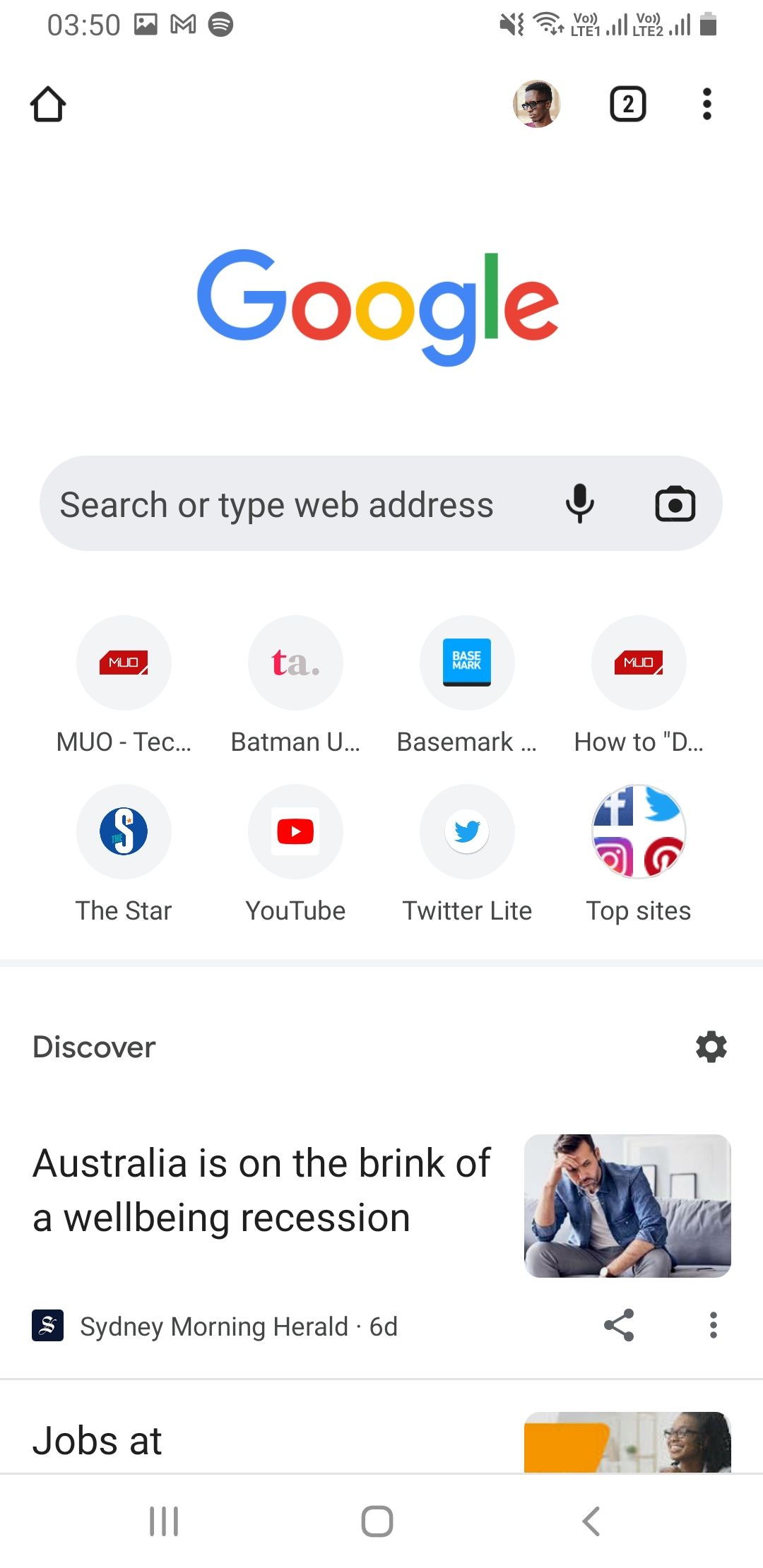A smartphone screenshot portrays the time as 3:50. The interface features a Google icon and a search box with the prompt "Search or type web addresses." To the right of the search box are a microphone and a camera icon. Below, there are two rows with eight oval-shaped app icons, each followed by abbreviated text labels. 

The top row includes:
1. An icon labeled "MUO-TEC..."
2. An icon labeled "Batman U..."
3. An icon labeled "Basemark..."
4. An icon labeled "how to D..."

The second row includes:
1. An icon labeled "the star."
2. An icon labeled "YouTube."
3. An icon labeled "Twitter lite."
4. An icon labeled "top sites."

A horizontal line separates these icons from the section below. Underneath, the screen displays the section labeled "Discover," accompanied by a gear icon. Further below is a news headline: "Australia on the brink of a well-being recession," attributed to "Sydney Morning Herald," dated six days ago. The headline is accompanied by a share button, an ellipsis for more options, and an image of a man wearing a shirt and tie.